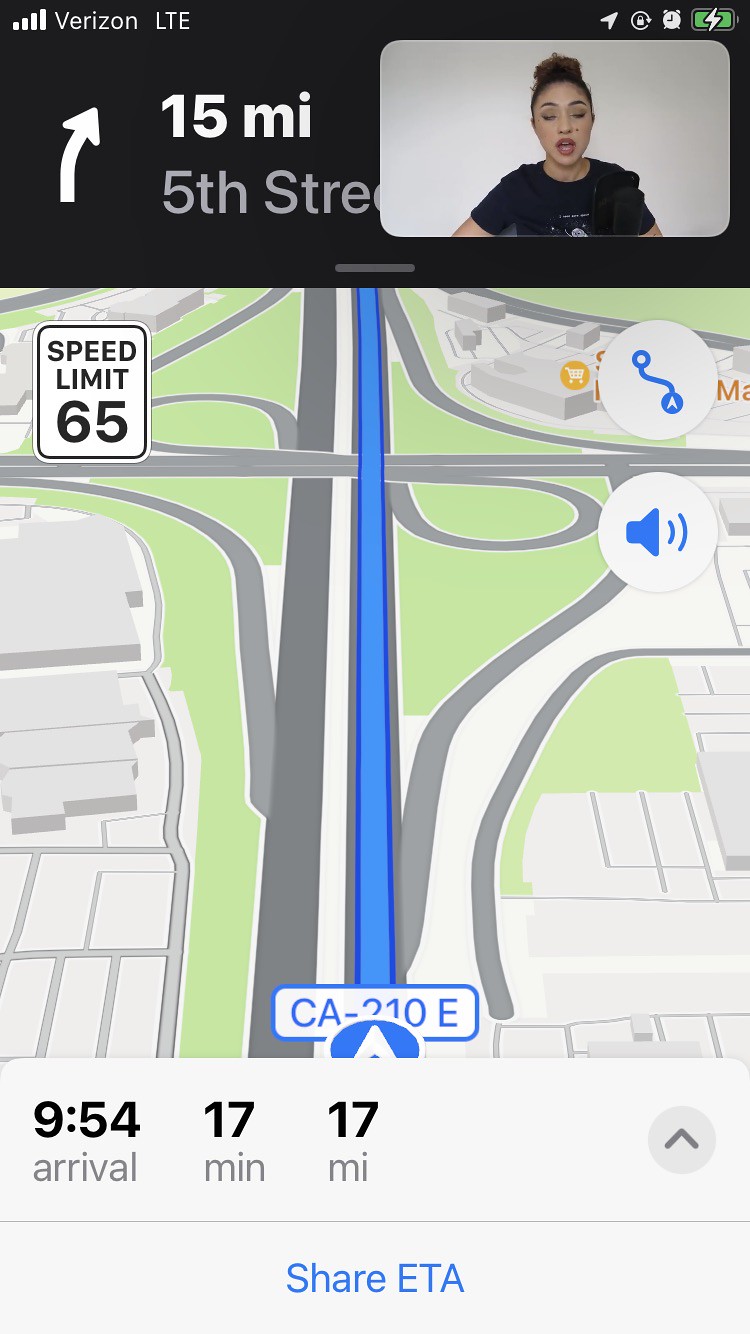**Detailed Descriptive Caption:**

This image appears to be a screenshot from a smartphone displaying a navigation application. Dominating the screen, the map shows a detailed layout of an interstate with visible on-ramps and off-ramps curving and looping around different roads. On the left side of the map, a speed limit sign prominently indicates a limit of 65 mph. Adjacent to the map, in the very top right corner, a small video is playing featuring a woman with dark hair styled in a bun, wearing a dark T-shirt. The video has a light gray background, and the woman, who has fair skin, appears to be speaking, although there are no additional visual cues to suggest the video's content.

Above the main map, a black bar from the app provides navigational instructions. An arrow to the left of the video icon indicates a rightward curve with text displaying "15 mi" and partially obscured "5th Street" with only "5th Stre" fully visible. Below this black bar, the map provides further navigation details, including the interstate layout and surrounding buildings or houses towards the bottom of the screenshot.

At the bottom of the screen, essential trip information is printed: the estimated arrival time, noted as "9:54", the distance remaining, "17 miles", and the time left to the destination, "17 minutes". Just below this information, there is a clickable link or button labeled "Share ETA," allowing the user to share their estimated time of arrival with others.